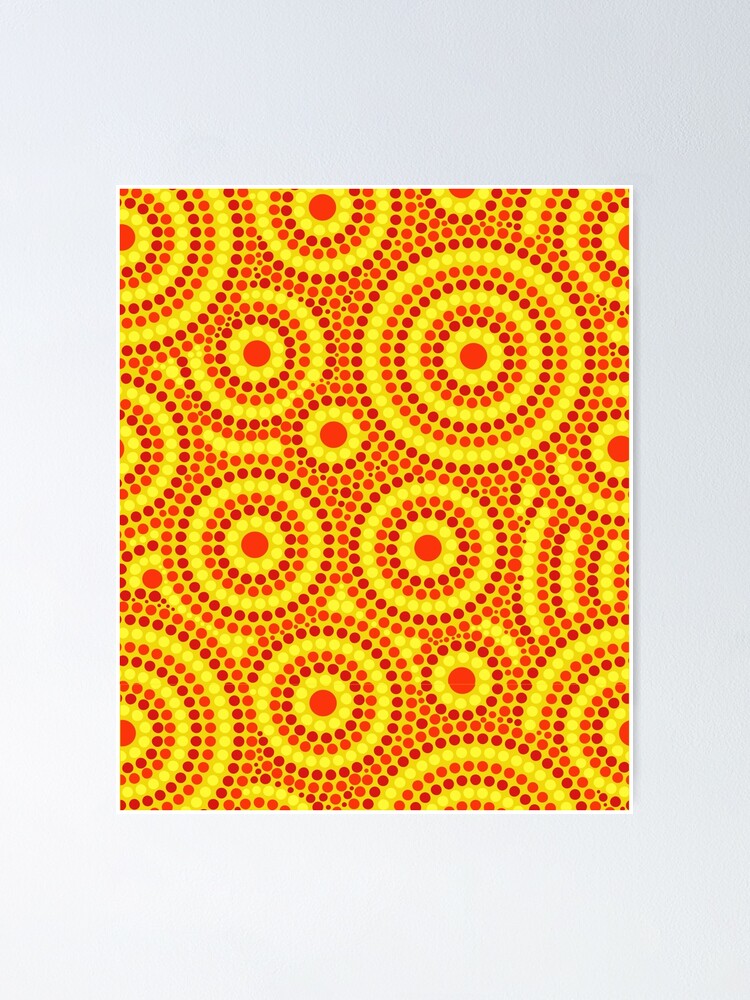The image is a vibrant and intricately detailed piece of mosaic tile art with a strong 60s, hippie-inspired aesthetic. Predominantly featuring a palette of bright yellows, oranges, and a gradient of reds, the artwork is dominated by a series of concentric circular patterns made up entirely of tiny seed beads. The central focus is a larger red dot, surrounded by layers of yellow, dark red, and bright red beads in repeating sequences. The composition showcases multiple circles, some with complex layering of up to five rings, others simpler with just one or two layers. Between these detailed spirals, spaces are filled densely with orange beads and accented with lines of yellow beads, creating a vivid, tightly packed pattern. The entire piece is framed by a white border against a light gray background, emphasizing its colorful, intricate design.